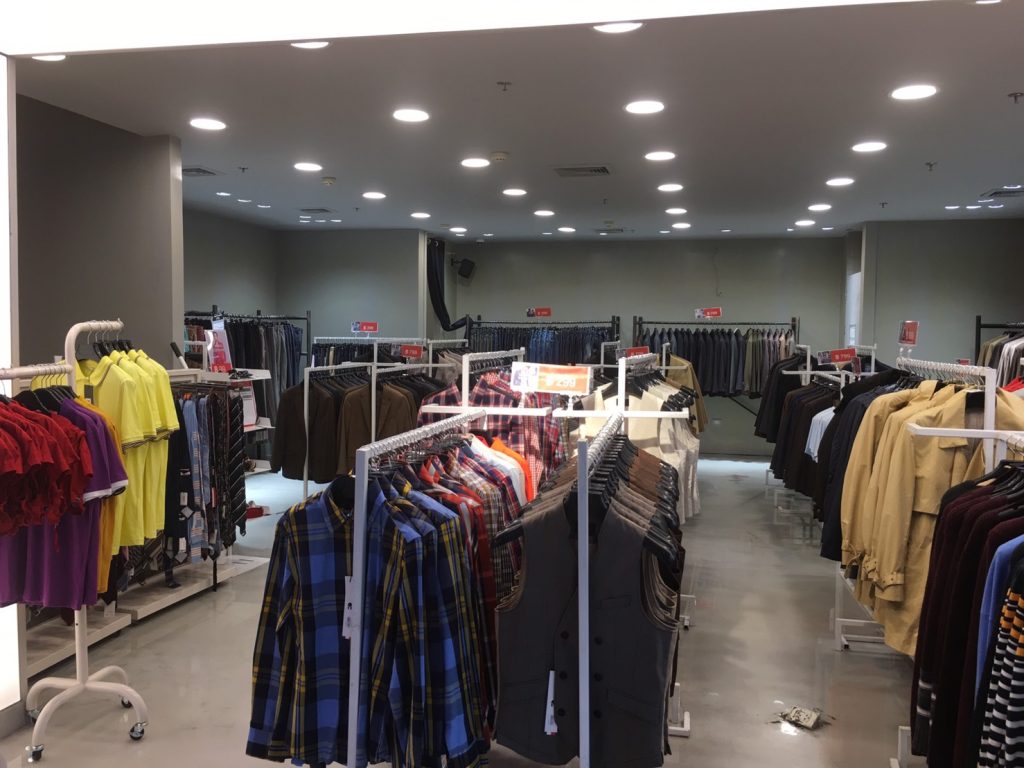The interior of this clothing store manifests a vibrant and well-organized space brimming with a diverse array of garments. On the left side, multiple racks display colorful shirts and blouses, showcasing a palette of red, yellow, and purple hues. Centrally positioned are racks dedicated to men's shirts with a rich variety of styles including flannels and vests. At the forefront of these racks, a blue and yellow flannel is prominently displayed, followed by a red and gray flannel, and a gray and pink one. Farther along are additional red flannels, a white one, an orange one, interspersed with more red options. The section on the right focuses primarily on vests in subdued beige and brown tones, blending seamlessly into an area dedicated to formal wear. This rightmost section houses an assortment of suit jackets, sport coats, and blazers. The store is bathed in bright, even lighting from numerous ceiling fixtures, ensuring the entire area is exceptionally well-lit. The immaculate and organized presentation of the store, combined with its modern lighting setup, suggests that it is a relatively new establishment.